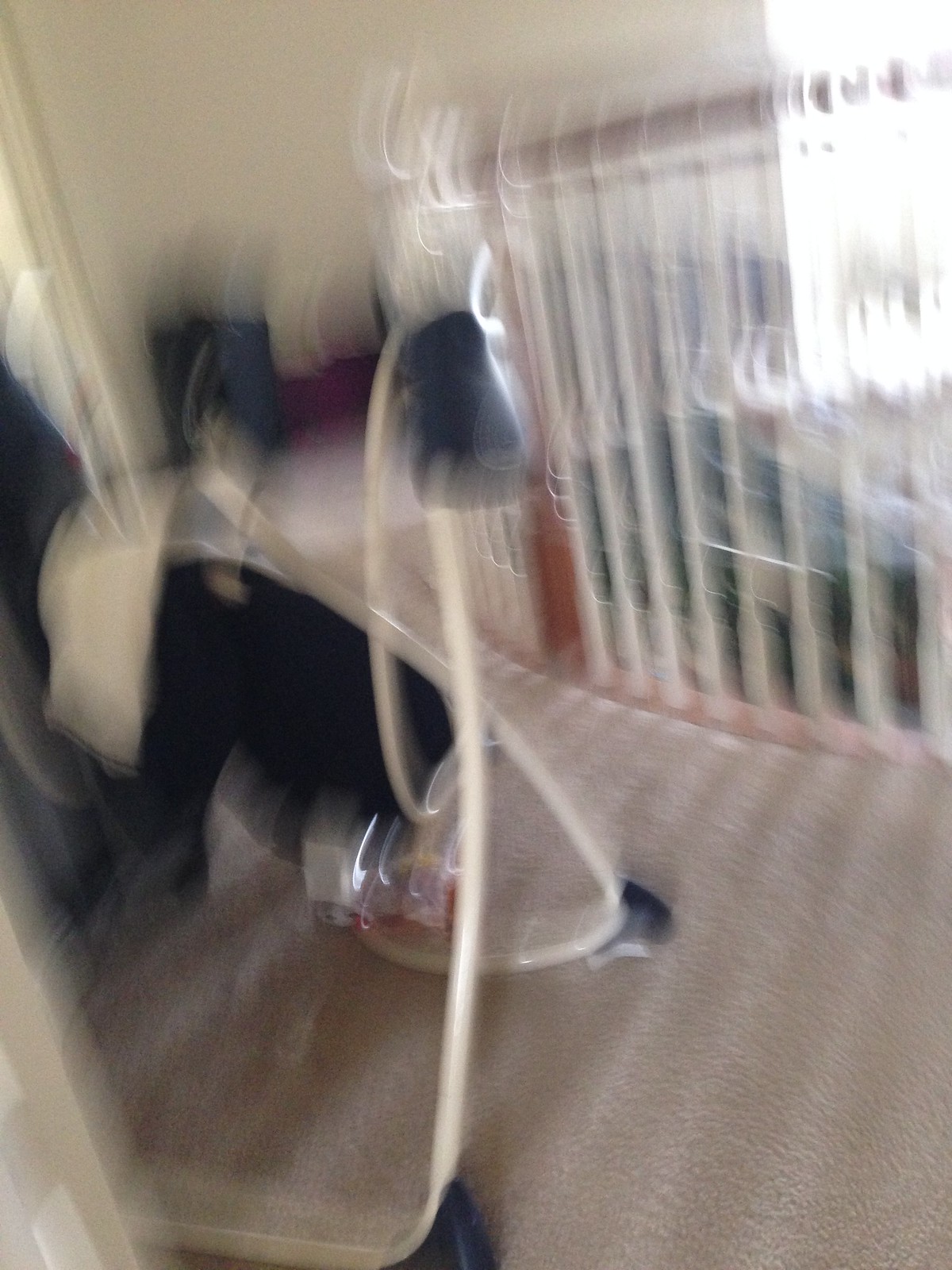This color photograph, taken inside a room, is somewhat blurred, making it difficult to discern precise details. The room features a beige carpet, on which rests a piece of equipment with a blue plastic component that connects to a white rod. This rod attaches to another blue part and extends into an additional white rod. A white gate, possibly part of a stairwell, is visible within the room. Sunlight streams in from a window, illuminating parts of the scene. The background wall is painted beige. There are indistinct blue items further back in the photograph, adding to the room's overall color scheme.